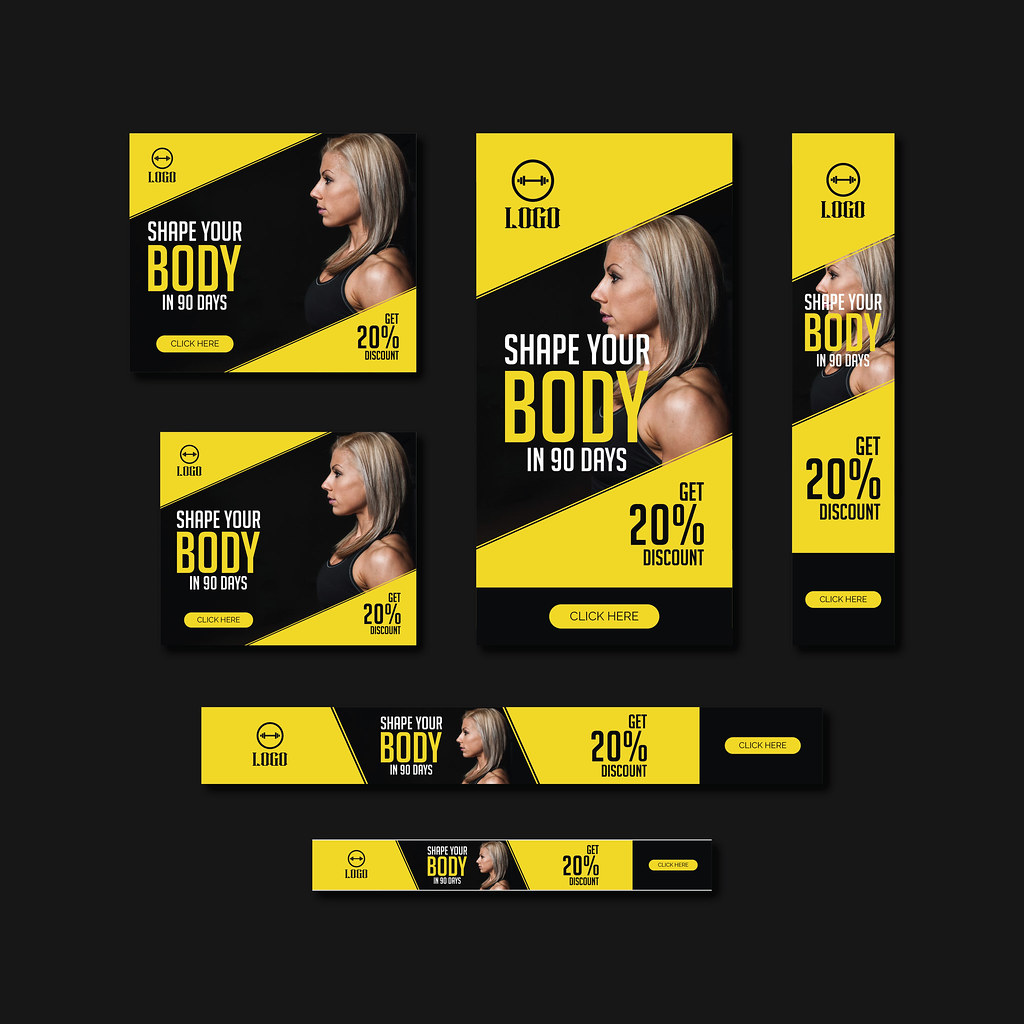The image showcases a variety of promotional materials for a product named "Logo" against a dark black background. These promotional elements feature a consistent design with a slanted yellow background and predominantly black accents, with white text complementing the visuals. The ads are distributed in various formats including square, vertical rectangle, and horizontal banner shapes. Each piece prominently displays a centered image of a blonde, tan woman, standing sideways and casting a serious look to her left, suggesting she's been engaged in fitness activities. Inscribed within each ad are the words "Shape your body in 90 days" and "Get 20% discount," with a "Click here" button on the right-hand side. The upper left corner of each material features the product's brand name "Logo", written in all caps with arrows pointing left and right. The comprehensive layout exemplifies a cohesive marketing campaign tailored to fit different digital ad spaces.